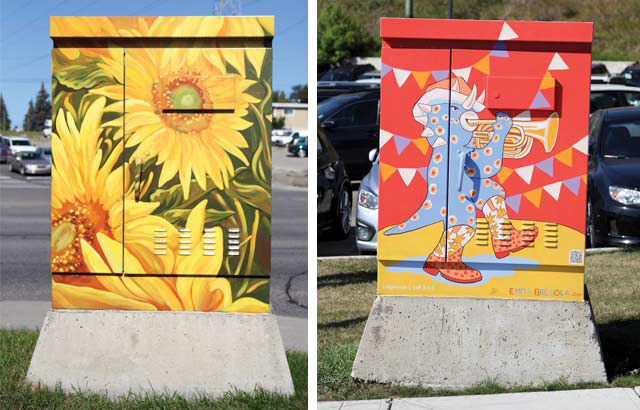The image is a two-panel photograph showcasing two distinct outdoor utility boxes adorned with vibrant murals, transforming these typically plain structures into eye-catching works of art. Both boxes, each perched on a concrete slab and placed in front of a parking lot under a clear, sunny sky, stand about five to six feet tall. 

The utility box on the left features an exquisite painting of large, bright yellow sunflowers with orange centers and green leaves, cascading over the green metal surface. The floral artwork almost makes the utilitarian nature of the box indistinguishable, blending it seamlessly with its urban surroundings.

Contrasting this, the utility box on the right boasts a whimsical depiction of a blue, horned dinosaur or dragon, adorned with yellow and orange spots. This quirky creature is dressed in yellow, red, and white cowboy boots and a peach-colored hat with a white brim, energetically playing a trumpet. The background enhances the playful theme, with circus-like pennants in white, blue, and orange hanging in the distance against a backdrop of red and black.

Both utility boxes contribute unique artistic flair to the urban landscape, standing as striking examples of how mundane city elements can be transformed into captivating visual experiences.